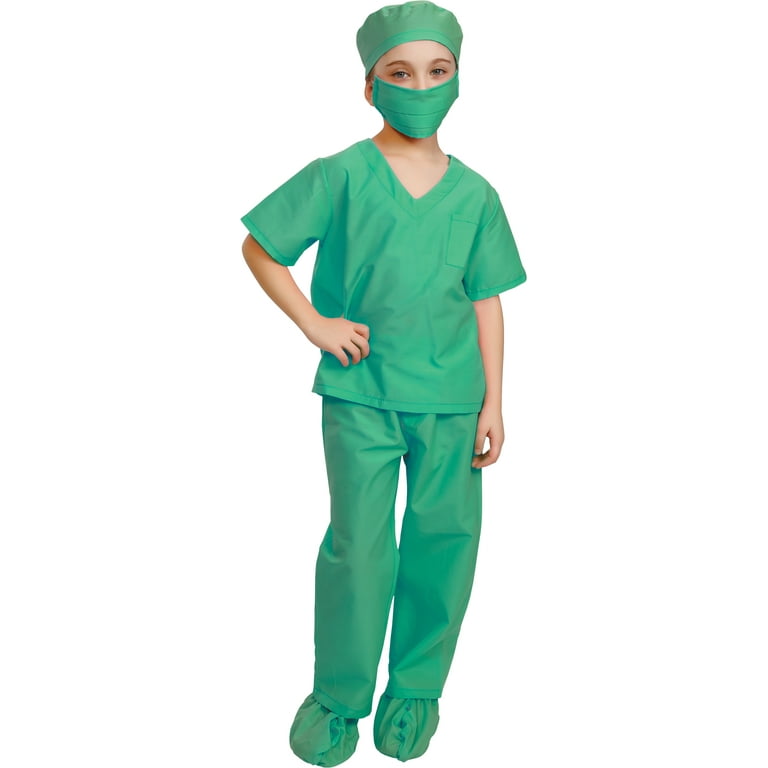The image features a young child, likely a little girl, dressed in a Halloween costume that resembles a nurse or doctor's outfit. Her attire is a cohesive seafoam green, including a cap that resembles a less-puffy chef's hat, a scrub-like top, and matching pants. She wears a coordinating green face mask that leaves only the area around her eyes visible, revealing her light-colored eyes and Caucasian features. Her right hand is placed on her hip, while her left hand hangs straight down. Instead of shoes, she has makeshift footwear resembling seafoam green trash bags tied up under her pant legs, blending seamlessly with the rest of her uniform. The background is a clean white, suggesting the use of a filter, and the image appears to be cropped, especially around her feet.